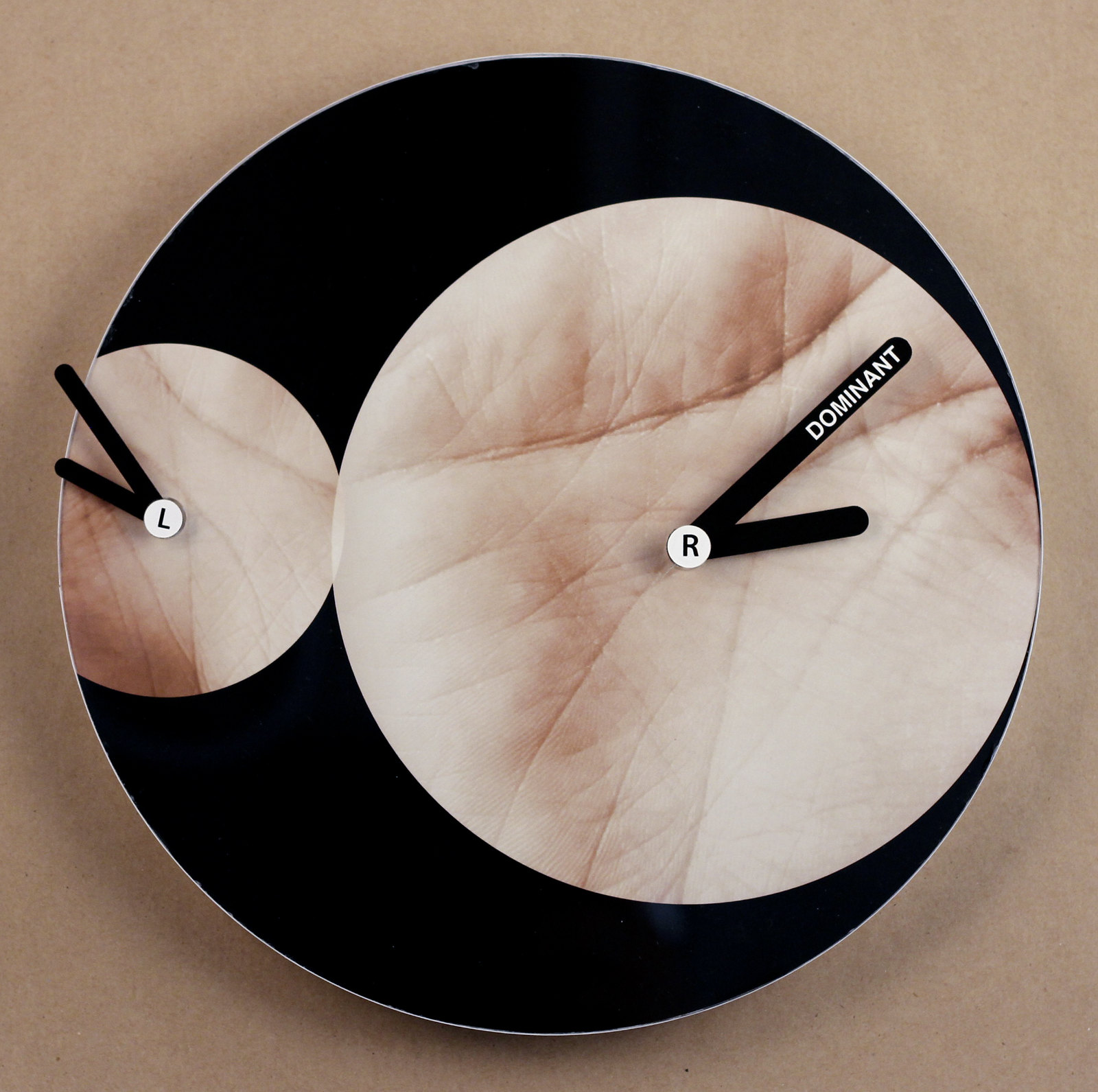This image features an abstract photo clock set against a tan or peach background. Dominating the layout is a large black circle with two smaller circles overlapping it – a small one on the left and a larger one on the right. The entire setup mimics a clock but with artistic elements. 

The smaller circle on the left showcases a detailed image of a palm. At its center is a white circle with a black "L," which is the hub from which two black clock hands extend; one long hand points up to the left, and a shorter hand is positioned slightly below it. The larger overlapping circle to the right also contains an image of a palm. Its center features a white circle with a black "R," serving as the base for two black clock hands. The longer hand here points up to the right, inscribed with the word "dominant" in small white letters, while the shorter hand is similarly placed below it. Both hands elements resemble traditional clock hands emanating from these central letters. A subtle silver border is visible on the left circle, adding a refined touch to this unique and intricate composition.